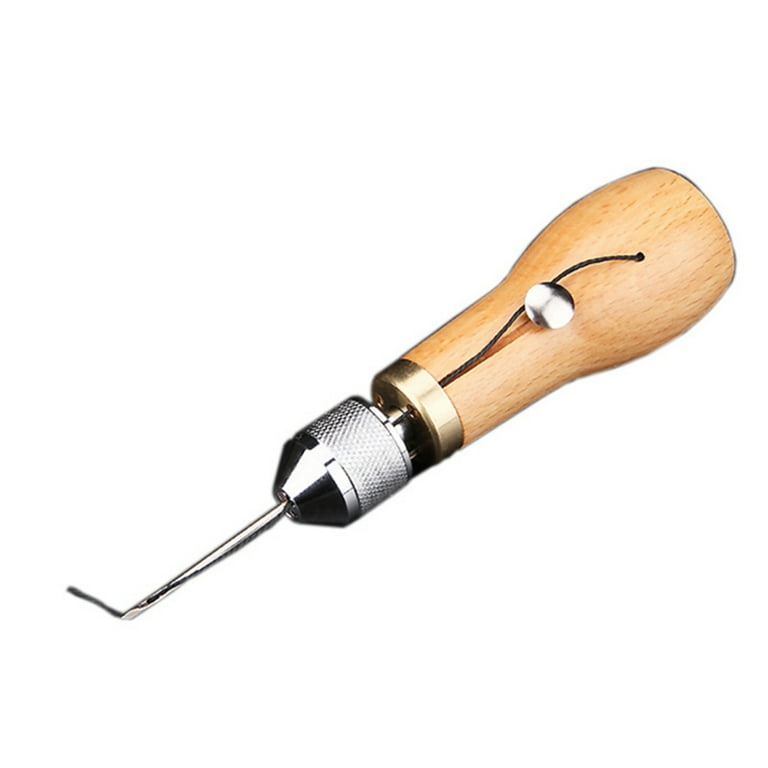The image depicts a specialized tool with a wooden handle and a distinctive, intricate design, set against a plain white background. The handle is approximately two inches long, crafted from brown wood, and features a gripping area that narrows from about an inch wide at the bottom to three-quarters of an inch at the top. Midway along the handle, there is a raised silver tack adorned with a piece of string wrapped around it. The end of the wooden handle broadens into a metallic cap resembling a lopped-off cone, which is reflective and grooved. Nestled within this metallic cap is a long, narrow metal piece that extends outward and bends at a right angle, forming an L-shape. This configuration suggests that the tool is designed for accessing hard-to-reach corners, possibly serving as a specialized instrument for woodworking or similar crafts. The entire tool is oriented at an angle running from the lower right toward the upper right in the image.